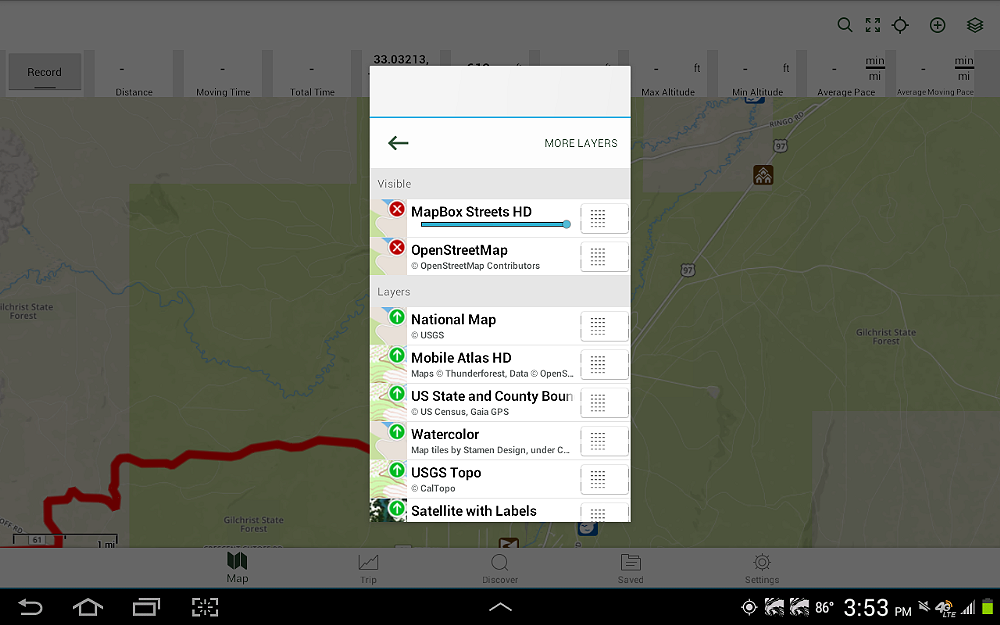Screenshot of a detailed map highlighting Gilchrist State Forest with several mapped locations. A prominent red line bisects the map, which features green, gray, and blue elements indicative of various terrains and water bodies. The map includes important markers like Highway 97, providing a clear route through the area. To the right, a pop-up window is visible, displaying several map layer options including "More Layers," "Map Box Streets HD," "Open Street Map," "National Map," "Mobile Atlas HD," "Thunder Forest Data," "U.S. State and County," "U.S. Census," "GPS," "Water Pillar," "Map Tiles by Stamen Design," and "USGS Topo." The diverse array of layers also includes "Cal Topo" and "Satellite with Labels," offering a comprehensive and customizable view of the region.